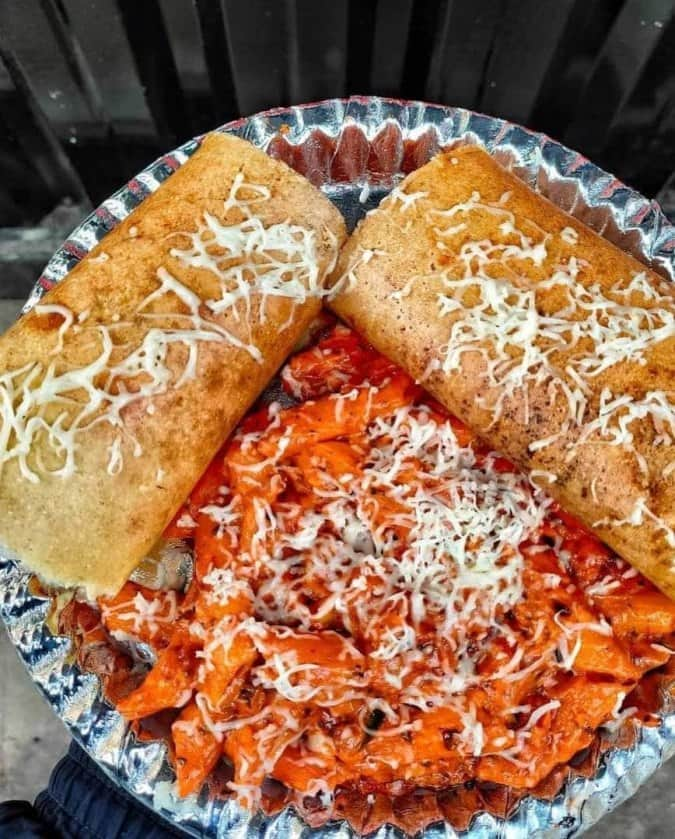This photograph features a vividly decorated circular plate, bordered first with blue and then red. Centered on the plate is a serving of ziti pasta, generously coated in a rich red sauce. The pasta is topped with fine shavings of white cheese, likely Parmesan or Romano, which impart a creamy, slightly nutty flavor. Flanking the pasta in the upper left and right sections of the plate are two tubular, burrito-like objects. These items resemble Indian parathas with their characteristic browned, flaky crust and are similarly dusted with the same white cheese. The unusual combination of Italian-style pasta and seemingly Indian-style stuffed parathas, both garnished with Parmesan, creates a striking and somewhat perplexing culinary juxtaposition.